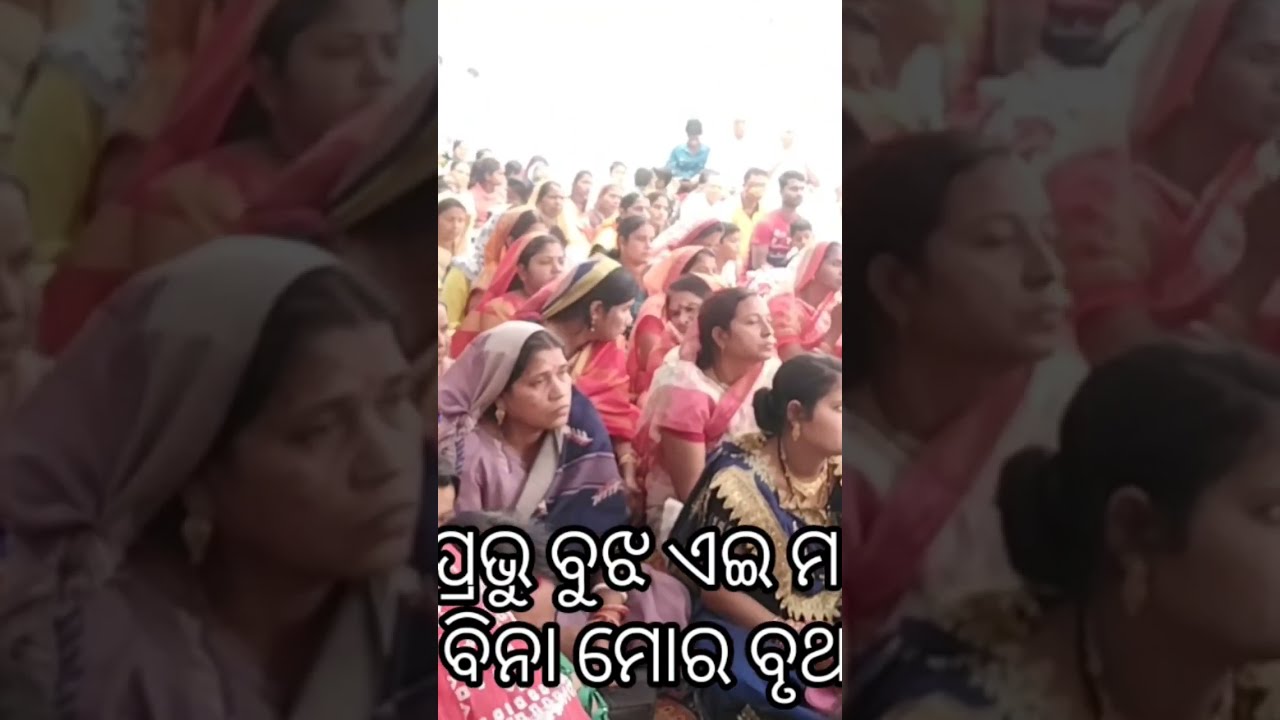The image is a horizontal rectangle divided into three equal vertical sections. The central section is clear and features a large group of people, predominantly women, gathered at what appears to be a party or a religious event. They are all colorfully dressed in traditional attire, with many wearing saris and matching headscarves. The women's dark hair is visible, and most are seated cross-legged on the ground, facing the same direction, possibly towards some focal point or activity that is out of frame. Some appear to be engaged in conversation. The background of the central section is washed out by light, making it difficult to discern any details there. Underneath the central image, there's text in a white, ornate script of an unidentified language.

The left and right sections of the image are blurred. On the left, there is a close-up of one of the women's faces from the central section. She is wearing a white headscarf and has a serious expression. The right section also showcases some part of the event but less clearly. Although the crowd primarily consists of women, a few men are visible in the background, suggesting possible gender separation. The overall composition of the image draws focus to the cultural and communal aspects of the gathering.